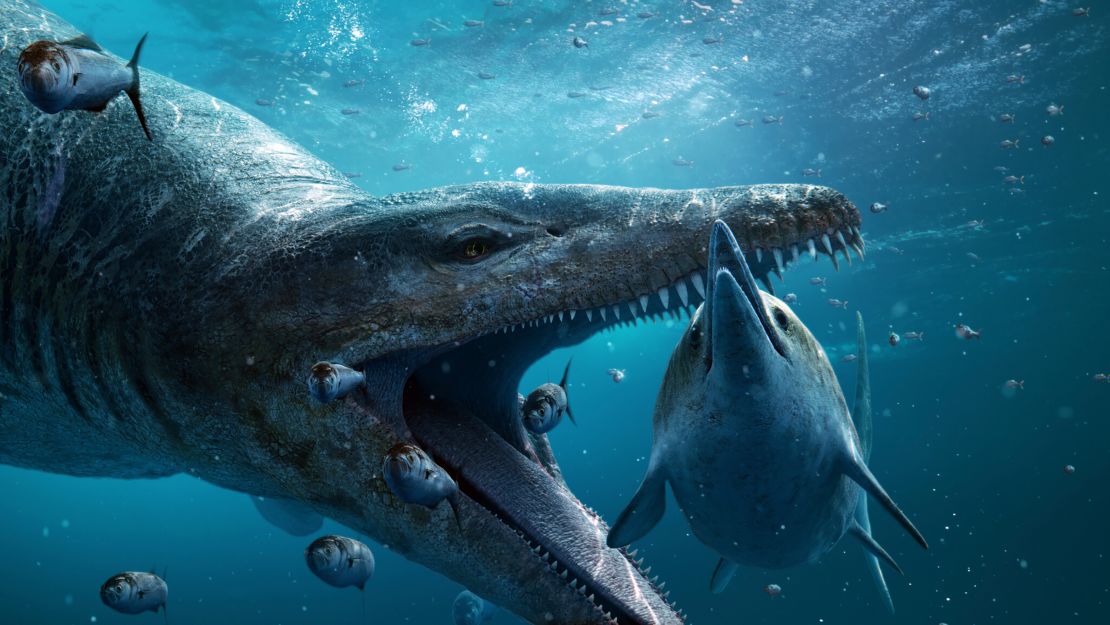In this vibrant underwater scene, an enormous prehistoric sea creature with shiny scales and razor-sharp teeth is depicted in a dramatic pursuit of a large, dolphin-like fish with a long, pointed beak and four flippers. The atmosphere is overwhelmingly blue, with bubbles dancing around that add to the tension. The illustration captures the moment just before the giant predator bites down on its prey, its angry expression menacingly contrasted against the frightened smaller fish urgently swimming away to escape their impending doom. The light filtering down from the surface adds an ethereal glow, and the surrounding silver and brown fish, which appear almost fantastical, accentuate the sheer size and ferocity of the ancient behemoth.